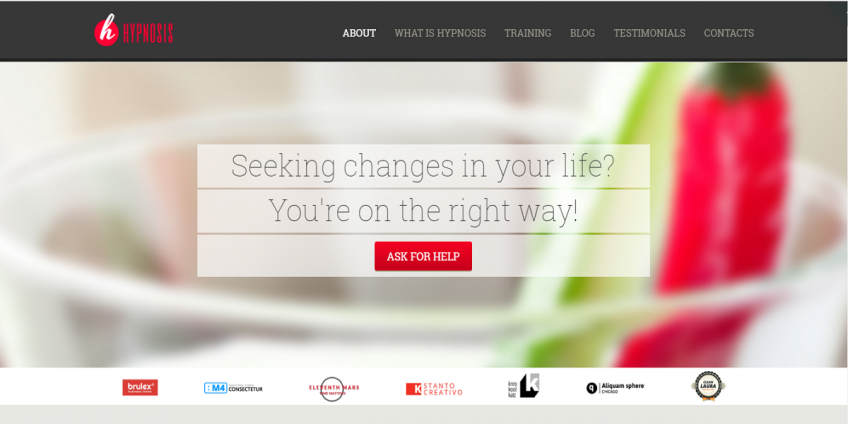This image is a screenshot from a website dedicated to hypnosis. The top menu includes buttons labeled "About," "What is Hypnosis?", "Training," "Blog," "Testimonials," and "Contacts." At the center of the page, a prominent message reads, "Seeking changes in your life? You're on the right way!" below which there is an "Ask for Help" button. The background image is slightly blurred but seems to feature a bowl or a glass filled with fruits and vegetables. At the bottom of the page, there are various logos: one for Brulex in red and white, an "M" for Consecutor, an Element Mars logo, "K" for Stancho Creativo, and another logo for Alaklamsphere Chicago.